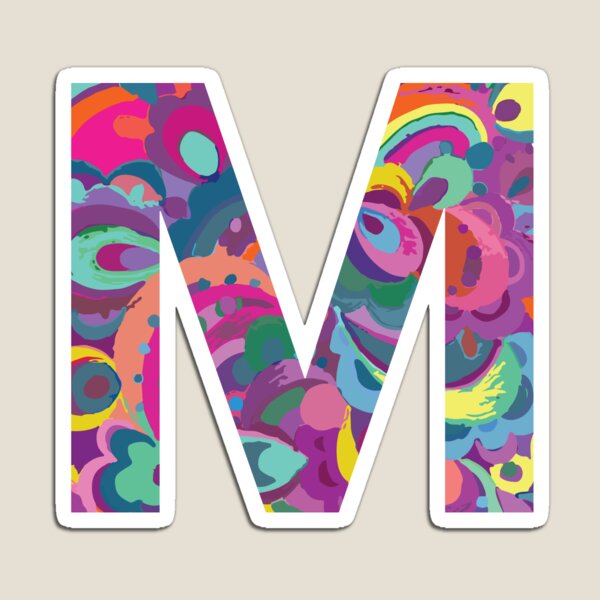The image features a large, capital letter "M" prominently centered on a square, beige background that resembles parchment paper. The letter "M" itself has a striking, three-dimensional appearance, emphasized by a simple white outline that creates a ridge effect against the background. The interior of the "M" is vividly filled with a psychedelic array of multicolored paint strokes, reminiscent of 1960s art styles such as the Sgt. Pepper's album covers or the playful aesthetics of the Yellow Submarine and Brady Bunch era. The colors within the "M" include a spectrum of shades such as purple, cyan, yellow, orange, pink, and green. These hues are applied in various forms, including circles, ovals, flower shapes, petals, and dots, creating an intricate, vibrant, almost kaleidoscopic effect that gives the letter an artistic and whimsical appearance.